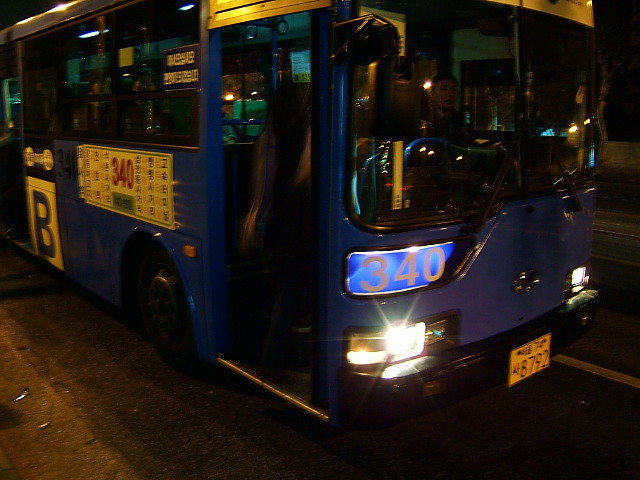This is a nighttime color photograph of a city transport bus in an Asian city. The image captures a three-quarter view from the side, showing the front of the bus where the door is located. The scene is dark, making subtle details hard to discern, but the bus's headlights and a nearby street lamp illuminate parts of the vehicle. 

The bus itself is primarily dark blue with yellow trim and a white roof. Prominent on the front is a lit panel displaying the number 340 in white letters on a bright blue background. This number also appears in red on the side of the bus along with a large "B" and additional Asian characters. The windshield is large and clear, revealing the driver, a male with short dark hair who appears to be of Asian descent. The bus has long rectangular glass windows down its side.

A yellow license plate with dark lettering is attached to the front of the bus. The bus is on a paved asphalt city street, adding to the urban nighttime ambiance of the photograph.